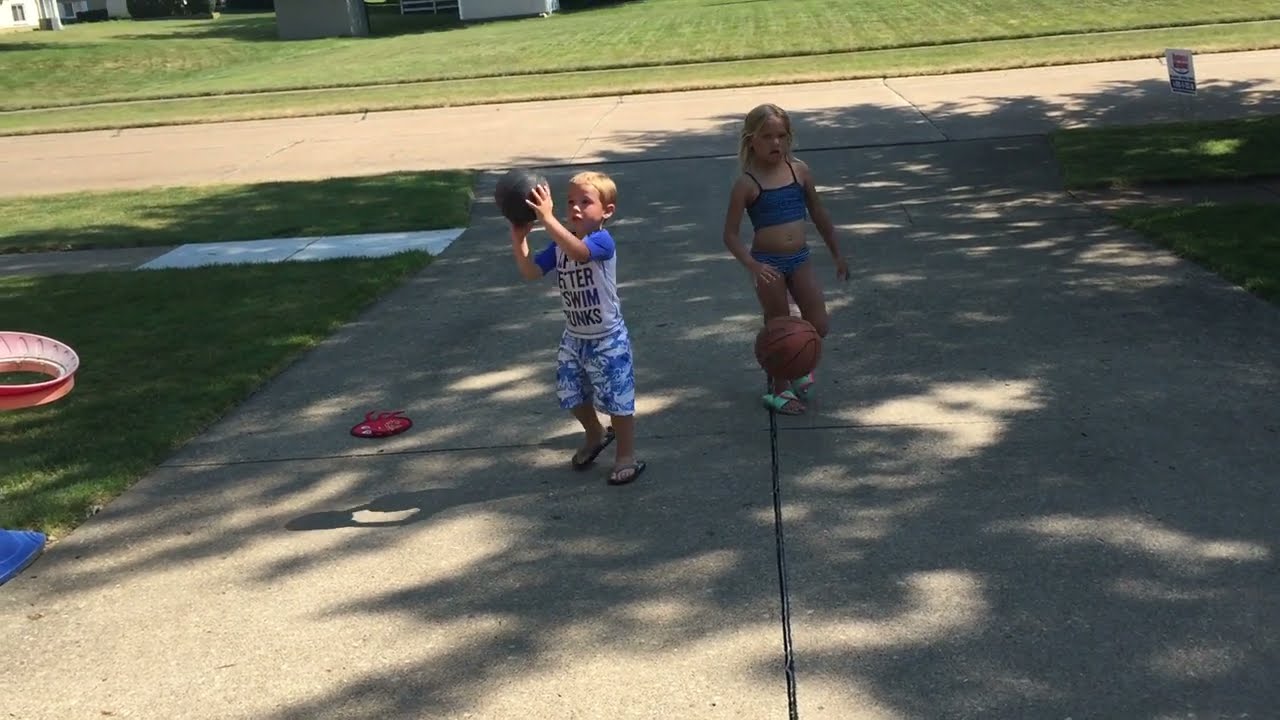In this vibrant, sunlit scene, two young blonde kids are captured in the midst of playful activity on their concrete driveway, set against the backdrop of a tranquil suburban neighborhood with well-manicured, verdant lawns. The older girl, slightly taller than the boy, is energetically dribbling a basketball. She is dressed in a blue swimsuit and sandals, radiating the carefree essence of a hot summer day. To her left, the boy is poised as if ready to shoot a ball, dressed in blue shorts and a white shirt adorned with unreadable lettering, paired with flip flops. The driveway merges into a sidewalk flanked by grassy expanses, and beyond, a quiet road with houses can be seen. Scattered toys on the lawn and the brilliant sunshine reflecting off the road and grass add to the lively summer atmosphere, suggesting a day full of outdoor adventures and possibly a refreshing dip in the pool later on.